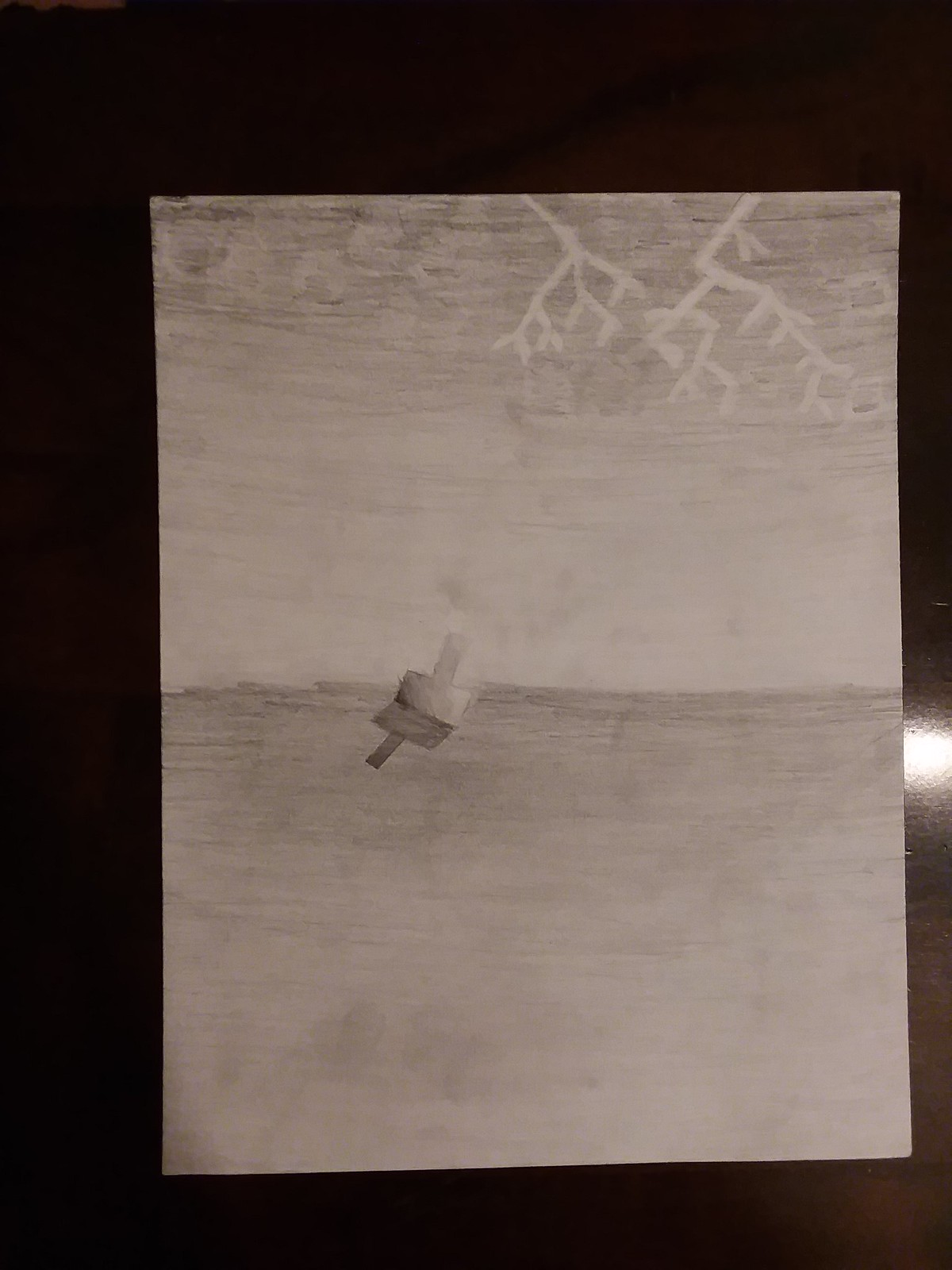A striking image captures Thor's hammer, Mjölnir, resting powerfully on the ground. Above it, the sky is alive with intense thunderstorms, with vibrant bolts of lightning slicing through the dark, tumultuous clouds. The electrifying scene, invoking the raw power and mystique of Thor, pays homage to the Norse god of thunder. The chaotic energy in the sky contrasts beautifully with the stoic, ancient weapon below, creating a dynamic and captivating composition.